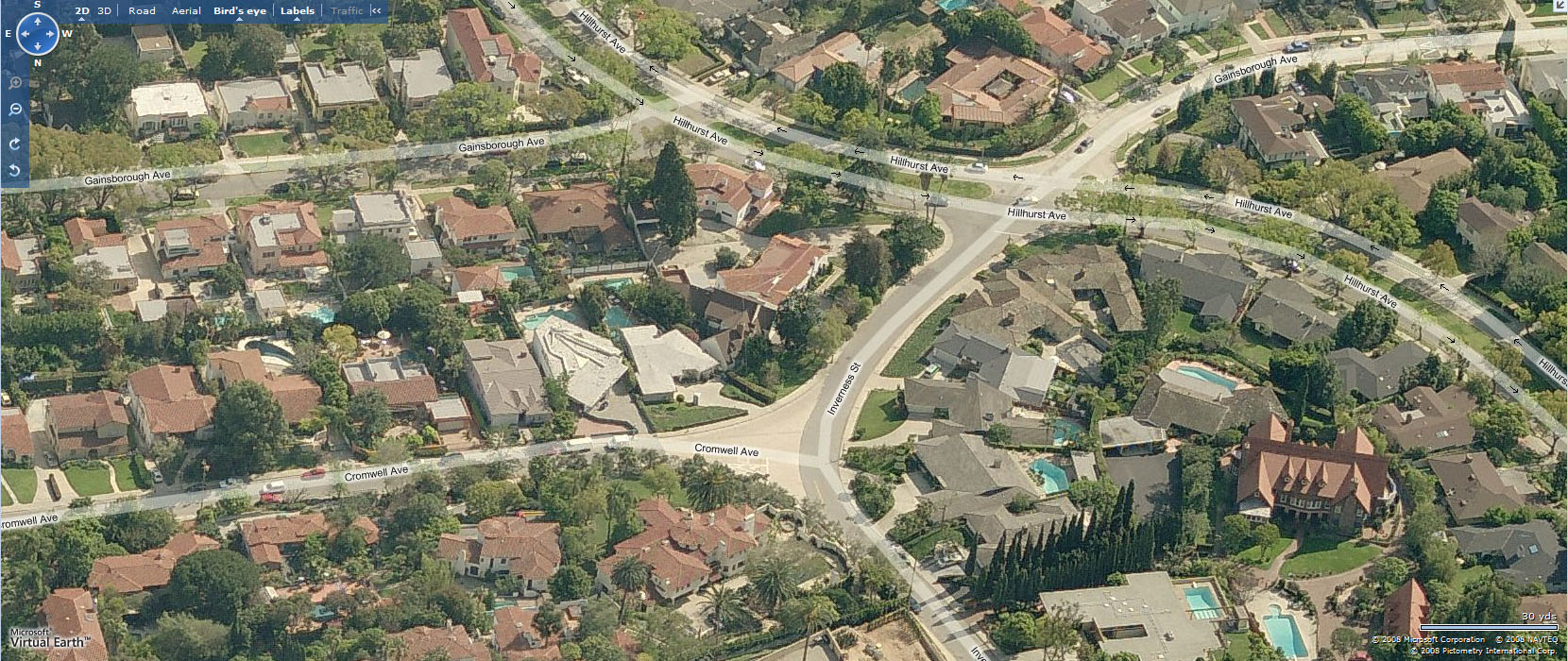An aerial daytime view showcases a sprawling, affluent neighborhood intersected by numerous streets, including Hillhurst Avenue and Inverness Street. The area features an array of grandiose houses, many reminiscent of mansions, characterized by meticulously tended landscaping. Numerous homes boast luxurious swimming pools and stately palm trees, further emphasizing the opulence of the locale. A white car is parked in front of one of the residences, while additional vehicles navigate the well-paved roads, completing the vibrant scene of a prosperous, well-maintained community.